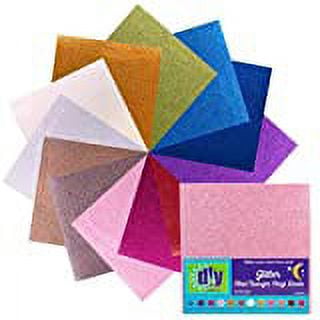The image features a meticulously arranged collection of colored squares, possibly made of tracing paper or tissue paper. Each square, about 4x4 in size, is arrayed in a star-like pattern, creating a visually striking display. The vibrant and varied colors include shades of blue, such as light blue and navy, as well as green, purple, pink, maroon, red, brown, tan, gray, and white. Some colors appear more than once in different shades, contributing to the rich, multicolored appearance. In the bottom right corner, there is a small section of text that reads “DIY” in blue lettering against a pink background, though the name of the company is not clearly discernible. The background of the image is white, emphasizing the vivid hues and delicate texture of the papers. Additionally, there is a small moon symbol visible in the bottom right-hand corner, adding a unique element to the intricate arrangement.